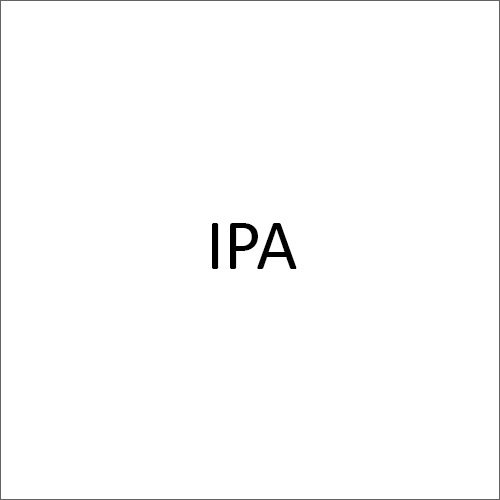The image portrays a minimalist design composed of a large white square with sharp edges and a thin black border. Positioned centrally within this white square are the bold, black letters "IPA," written in all uppercase. The font resembles Arial and is noticeably in a sizable font, potentially in the 30s. The background and the interior of the square are pure white, creating a stark contrast to the black letters and border. While "IPA" could represent various acronyms, it prominently suggests India Pale Ale, a notable type of hoppy beer, possibly indicating the label’s purpose in identifying this specific beer variety.